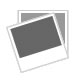This sepia-toned photograph captures an upright, partially-open book with two visible pages, suggesting the atmosphere of the old West. On the left page, a large black-and-white image shows a worn, tired-looking man with a long beard and a cowboy hat, standing next to a horse. The horse, which has distinct black spots on its nose and crown, stands close to the man with large, expressive eyes. The man is dressed in a dirty, tattered V-neck shirt, jacket, and wrinkled pants secured with a belt. A black strap crosses his chest. Behind them, a line of trees and patches of grass are visible, adding depth to the backdrop. The text above and below this image hints at its historical content.

On the right page, the layout includes text with two prominent titles: "Muzzle-Loading" and "A Practical Hunting Gun." The center of the page features a medium-sized black-and-white photograph of two men on horseback near a large body of water, amidst a sandy terrain. One man wears a black hat and coat, while the other, seen from behind, is in a fur hat and vest. Both are seemingly trying to guide their horses to drink, adding a dynamic element to the scene. Text paragraphs are placed above and below this image, hinting at the narrative content surrounding these vivid depictions.